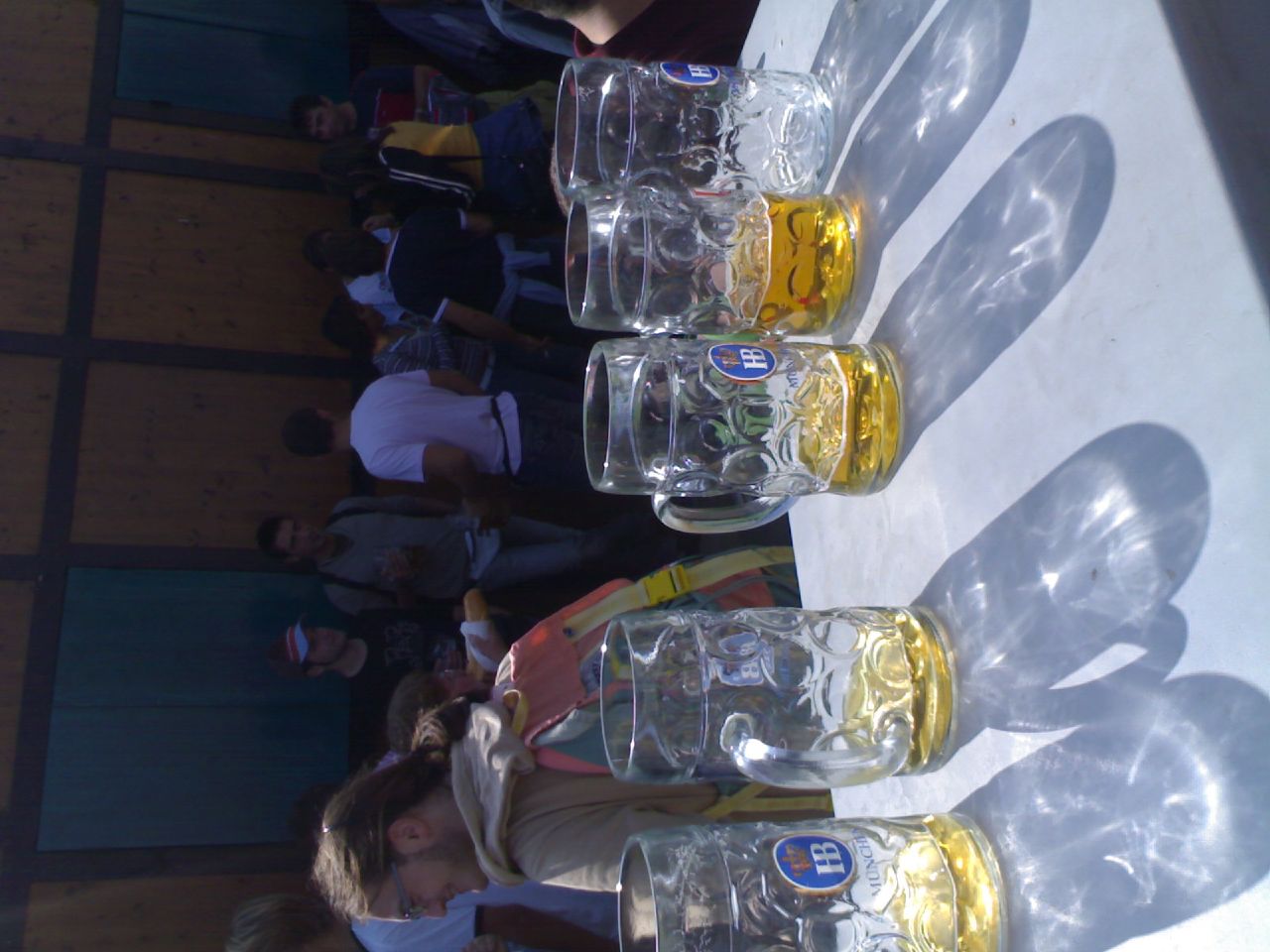In this detailed image, which has been turned 90 degrees counterclockwise, we see a row of five beer mugs on a gray counter. The first four mugs from the left contain a small amount of amber-colored liquid at the bottom, while the fifth mug is empty. Each mug features a blue circle with the number 18 inside of it. The scene is set at an outdoor event on a sunny day, as evidenced by the bright sunlight casting intricate, sparkly shadows through the clear glass of the mugs.

In the background, behind the beer mugs, stands a man wearing a brown hooded sweatshirt and an orange and yellow vest or backpack. He has a ponytail and appears to be engaged in conversation. Further back, a group of at least five or six other people can be seen, including a man in a white t-shirt. They are gathered near a wall that is accented with blue and brown sections and black dividing lines, creating a distinct backdrop. The focus of the image is the beer mugs, but the vibrant activity and people in the background provide a lively context to the scene.